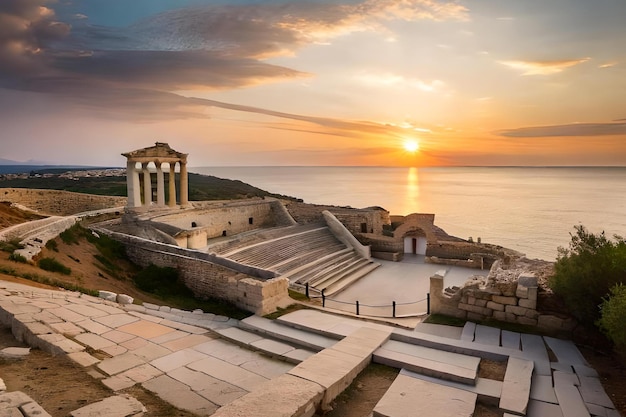This landscape photograph captures a breathtaking sunset over a calm ocean, with the sun positioned just above the horizon in the center of the image. The sky showcases a gradient of colors, transitioning from the soft blue at the top to vibrant oranges and yellows around the setting sun. Reflecting the sunlight, the tranquil water mirrors the serene beauty of the sky above.

In the foreground, the picture features an ancient Greek amphitheater carved from stone. The well-preserved structure exhibits tiered stone seating curving around a flat stage area. The amphitheater is partially bordered by a distinct wall that separates it from the ocean. To the side, a cluster of five circular columns stands, hinting at the grandeur of Greek architecture, and possibly made of marble or granite, with an A-frame roof structure partly visible.

Further right, some greenery provides a verdant contrast to the grey stone ruins. In the distance, towards the left-hand section, there are hints of civilization marked by patches of white, suggesting towns or buildings dotting the landscape. This photograph beautifully blends natural splendor with historical intrigue, evoking a sense of timelessness and cultural heritage.